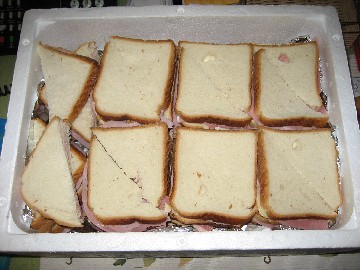The photograph is a close-up shot of a rectangular, white styrofoam container, possibly a cooler, filled with sandwiches. The container, which has a deep recess and aluminum foil lining the bottom, is placed on a white paper surface. The sandwiches are made with white bread that has a dark brown crust and are filled with pink meat, likely ham, which slightly protrudes from the edges. The left side of the sandwiches is neatly organized: the wedges are cut diagonally and stacked on top of each other in opposite directions. The remaining sandwiches are arranged in two horizontal rows and four vertical columns, with each sandwich split into triangles. The background consists of a desk, but the focus of the image remains tightly on the container and its contents, leaving little visibility of anything else outside the container.